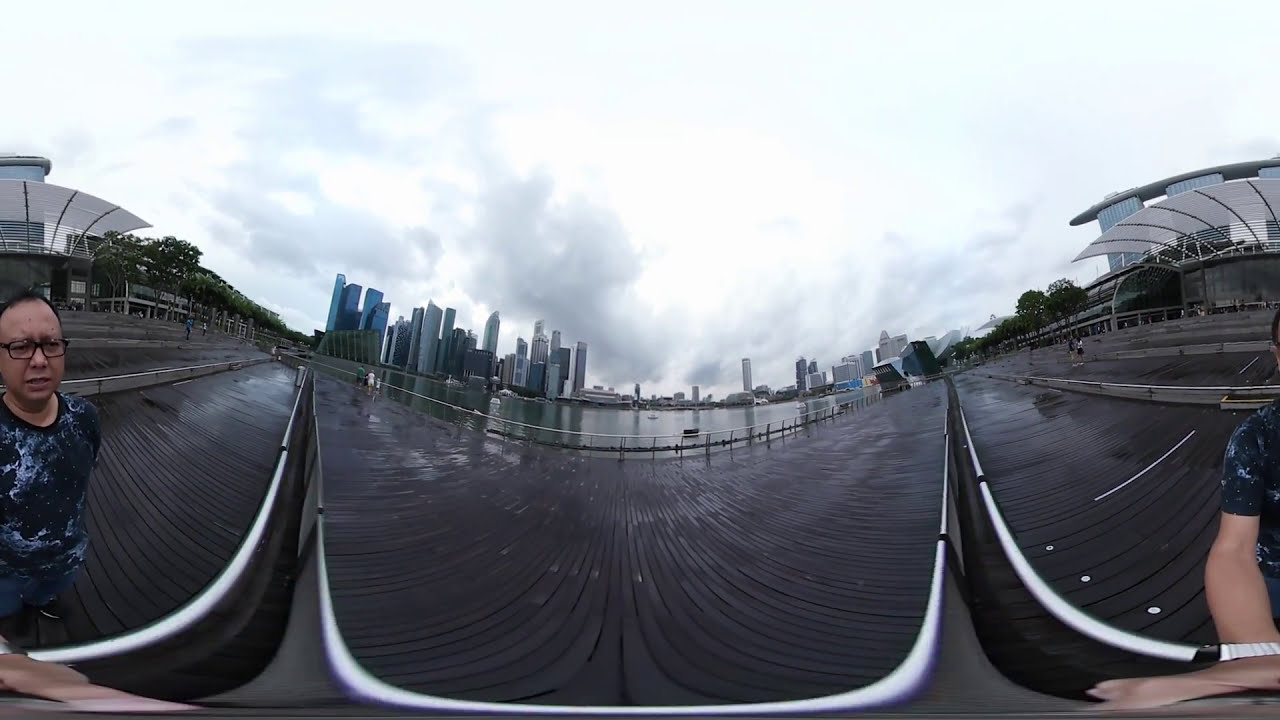This photograph showcases a panoramic view of a boardwalk that splits and wraps around a body of water, creating a dynamic, sweeping perspective. In the foreground, a woman, whose gender is initially ambiguous but appears to be female based on further context, stands on the boardwalk wearing a tie-dye blue shirt, black glasses, with her hair pulled back. Portions of her figure are visible on both the left and right sides of the image, hinting at a 360-degree or distorted, photoshopped view. In the midground, you can see a railing, and the dark brown, possibly wet boards of the walkway suggesting recent rain. The background features a serene lake dotted with several boats, extending towards a striking city skyline. Multiple skyscrapers dominate the left side of the skyline, including a cluster of four blue towers, while gray and silver buildings extend further right. The sky is overcast, filled with varying shades of gray clouds, adding a reflective, silverish quality to the scene. Overall, the photograph captures an urban landscape juxtaposed with natural elements, encapsulating a moody and reflective atmosphere.